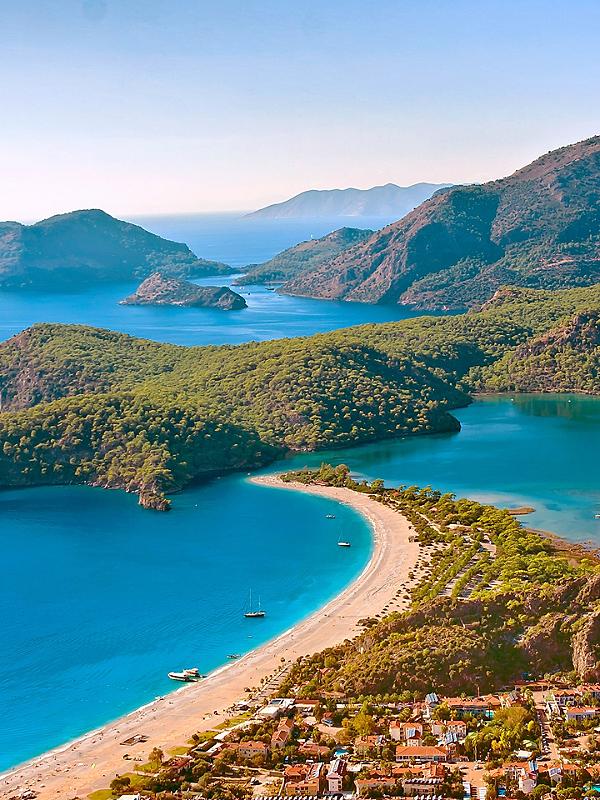The picture vividly captures a stunning coastal scene, suggestive of a Mediterranean locale, possibly Italy or France. The image, taken from an aerial perspective, shows a pristine, bright blue sea stretching out towards the horizon with a few boats and yachts dotting the water. Anchoring the foreground is a long, curving beach with white sand, leading to a settlement characterized by terracotta-roofed houses typical of Mediterranean architecture. Forested hills flank the coastline, creating a lush green backdrop that rises semi-mountainously. Further in the distance, a tiny island surrounded by water can be seen, also adorned with boats, while a grand, forested mountain looms on the right. In the hazy background, a solitary mountain extends into the vast body of water, enhancing the scenic beauty of the place. The scene is bathed in bright sunlight, suggesting a warm, clear day, with minimal signs of human activity, making it appear tranquil and almost idyllic.